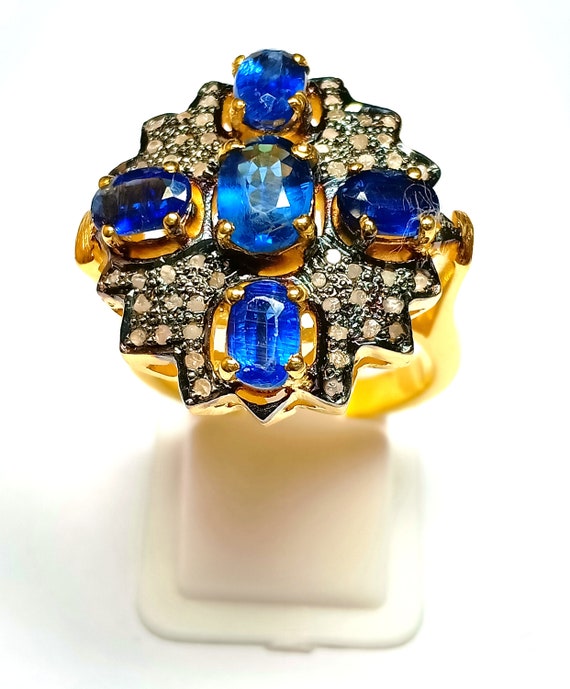This is a highly detailed portrait-mode image of an extravagant gold ring, possibly mistaken for a pin due to its angle on a cream-colored, foam ring holder with a square base and an upward pointing triangle to support the ring. The ring is the central focus and features an array of five bright blue sapphire-like gems arranged in a cross pattern, with the largest gem at the center and four smaller ones situated at each cardinal point. These ocean-blue stones exhibit remarkable shine and possibly contain images, suggesting a digital enhancement. They are beautifully inlaid in a gold setting, which also incorporates a mix of black, grey, and silver elements that form a striking petal-like background, contributing to the overall luxurious and intricate appearance. Surrounding the sapphires are smaller, sparkling gems that could be diamonds or cubic zirconia, adding an extra layer of brilliance. The entire composition is brilliantly lit, highlighting the shimmering quality of the metals and stones, against a pristine white background with a subtle shadow at the bottom, further enhancing the ring's elegant presentation.